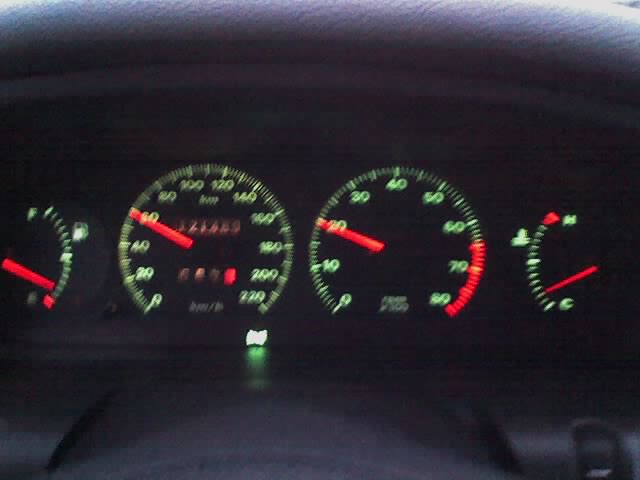This image captures a close-up view of a car’s dashboard, highlighting an array of gauges and indicators with intricate detail.

On the far left is a fuel gauge, designed in a semi-circular shape. This gauge features an 'F' (representing Full) at the top and an 'E' (for Empty) at the bottom, with several dash marks in between to indicate fuel levels. Notably, there is a red dash mark by the 'E', signifying a critical low fuel level, and a small gas tank icon next to it. The gauge’s red needle is pointing close to the red mark, suggesting the fuel tank is almost empty.

Adjacent to the fuel gauge is a larger, almost complete circular dial—this is the speedometer. The speedometer is marked with numbers ranging from 0 to 220, in increments of 20. The red needle on this gauge points just below the 60 km/h mark, indicating the current speed of the vehicle. Embedded within the speedometer is an odometer, displaying six rectangular slots with numbers that are not clearly readable. Below it, there appears to be a trip meter, which also has four rectangular slots with indistinguishable numbers. Additionally, a green symbolic icon, possibly a warning light, is visible beneath the speedometer.

Continuing to the right, another large circular gauge similar in size to the speedometer accommodates the tachometer. It is marked with numbers from 0 to 80, incremented by 10. Sections from 65 to 80 are colored in red, while the rest of the gauge is in green, indicating safe and unsafe engine revolutions per minute (RPM). The red needle here rests at 20, suggesting the current engine RPM.

On the far right, there is a quarter-circle temperature gauge, characterized by an 'H' (for Hot) at the top and a 'C' (for Cold) at the bottom. Red tick marks near the 'H' highlight dangerous temperature levels, while the rest of the scale is in green. The red needle on this gauge points slightly above the 'C', suggesting the engine temperature is relatively cool.

This detailed and descriptive image of the car’s dashboard offers a comprehensive view of the critical informational displays vital for vehicle operation.